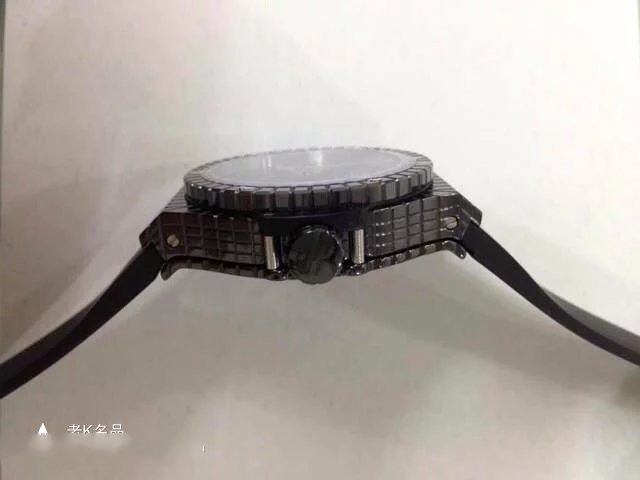This black and white photograph showcases a detailed side view of a watch, emphasizing its intriguing textured design. The side of the watch features a unique pattern of small, box-like structures that break away from a solid metal appearance, adding depth and visual interest. Prominently displayed is the adjustment dial, complete with fine cutouts around its circumference, hinting at precision engineering. The side of the watch is fastened to the main body with visible screws, adding an industrial touch. The watchband appears to be quite flexible, demonstrated by a slight bend, and the overall watch surface carries a dark hue, resembling a dark brown or gunmetal shade. Additionally, the photograph captures the watch glass and a touch of Asian script in the lower left-hand corner, suggesting a cultural element to the timepiece. All of this is set against a light gray background, which contrasts with and highlights the intricate details of the watch.